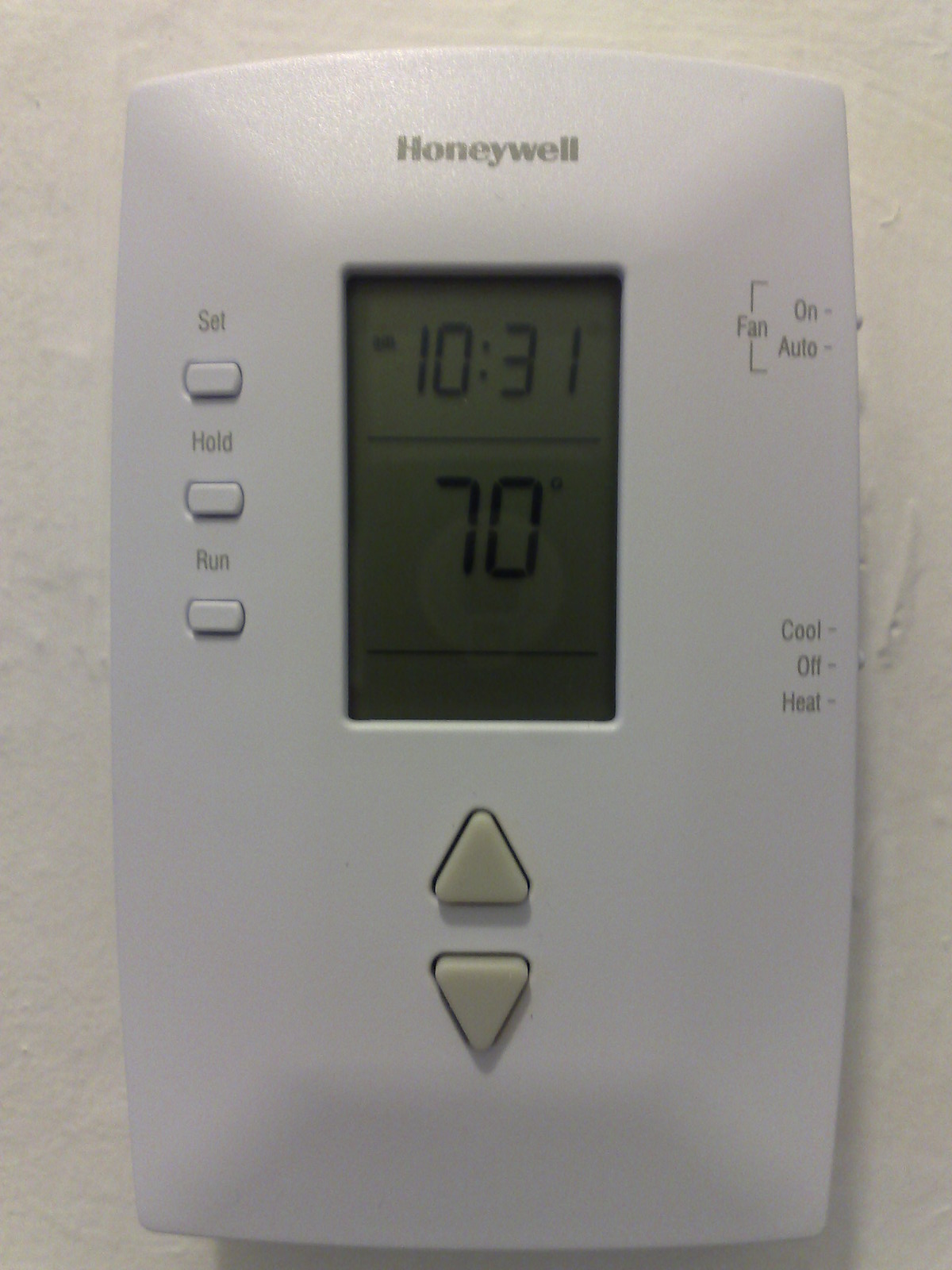Indoor, color close-up photograph of a Honeywell brand digital house thermostat mounted on a white wall. The rectangular device features a dimly lit LED display in the center of the upper portion, clearly indicating the number "1031" in digital figures. Below this, a horizontal line separates the main display from a reading that shows "70 degrees," followed by another horizontal line.

To the left of the display on the white thermostat case, there are three oval-shaped white buttons. The top button is labeled "SEL," the middle one says "Hold," and the bottom one is marked "Run." Below the LED display, two off-white rectangular buttons are positioned, one pointing upward and the other downward.

On the right side of the LED display, towards the upper right portion of the housing, the word "Fan" is visible, followed by the options "On -" and "Off -." About an inch below, words "Cool -" "Off -" and "Heat -" appear, with small protruding buttons near these labels.

Above the display, the brand name "Honeywell" is printed in gray letters. The image is well-focused, though dimly lit, with the primary light source appearing to originate from above, creating a lighter upper section and a darker lower section. No other text or print is visible in the image.